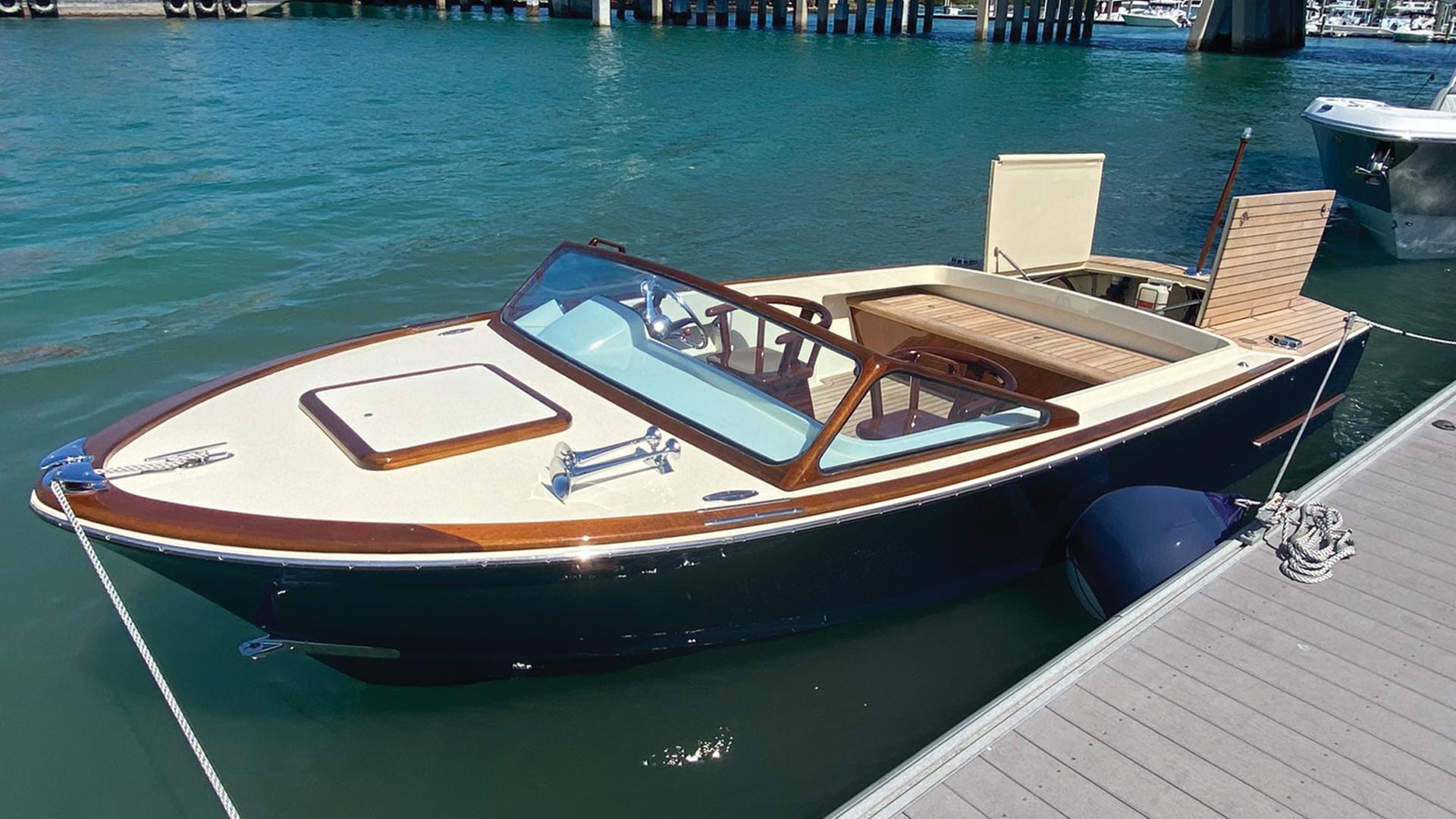This is a detailed color photograph of a sleek, small, dark blue motorboat moored next to a grayish-white floating dock in a tranquil harbor with dark turquoise water. The boat's lower hull is dark blue, transitioning to a cream-colored top accentuated by dark wooden trim. At the front tip of the boat, which is positioned towards the left side of the photo, there is a visible mooring point. Protecting the steering wheel area, which has light blue accents, is a small glass pane. 

The deck features two dark wooden captain’s chairs and a lighter wooden bench at the back, all arranged for comfort and functionality. Two hatches at the rear are raised, presumably providing access to the storage compartments and the motor. The boat is securely tied to the dock, with an additional mooring anchor attached to a cleat in the bottom right-hand corner of the image. 

Behind this boat, a portion of another white and blue craft is visible. The serene background showcases support posts for a bridge, along with distant boats dotting the horizon, lending a sense of depth and context to this harbor scene. The absence of people and animals, combined with the sunlight illuminating the scene without any visible writing, adds to the calm and orderly atmosphere of the photograph. A buoy is strategically placed between the dock and boat to prevent damage.